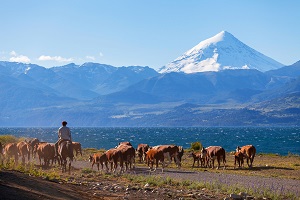The photo captures a dynamic scene set in a vast, rugged landscape. In the foreground, a man on a white horse is herding a group of about a dozen cows along a grayish gravel road, which might also be considered a dirt path. The road is flanked by some sparse greenery. This setting stretches out across what appears to be a prairie or valley that leads towards a stunning backdrop of rugged, non-snow-capped mountains. Dominating the scene, however, is a striking, tall, pyramidal snow-covered peak that looms over the other smaller hills and mountains. The sky behind this impressive triangular mountain is a light blue, scattered with a few clouds. The nature of the space between the foreground and the mountain range is ambiguous; it could potentially be a body of water or simply darker land, suggesting the shore of a large lake that spans the middle section of this photograph.